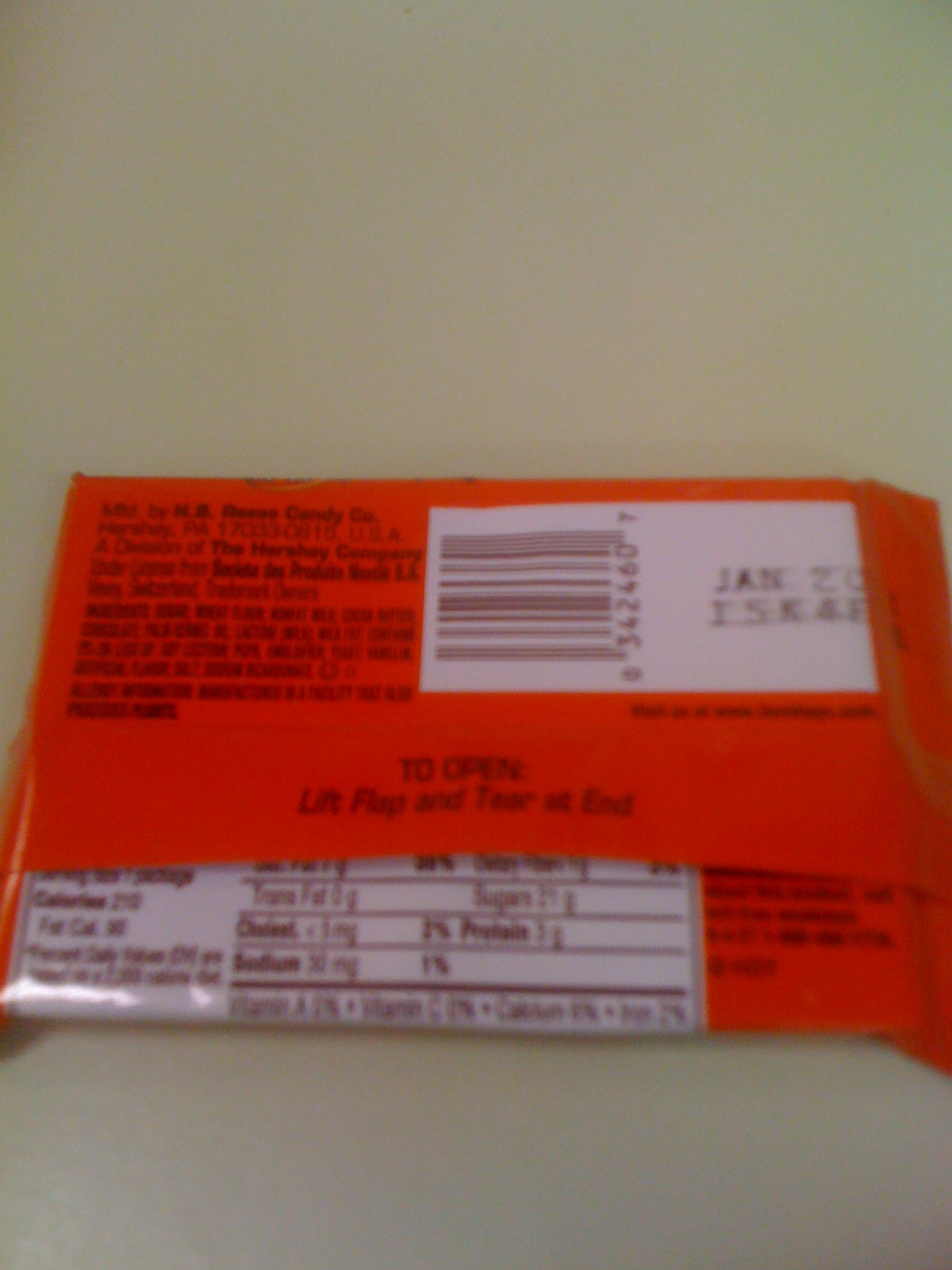Here is a detailed and cleaned-up caption for the image:

"A red candy wrapper from the Reese Candy Company, featuring a partially visible white rectangular barcode area at the top. The barcode section also shows an expiration date cut off at 'January 20'. Below the barcode, additional numbers are visible. To the left of the barcode area, text in black indicates that the candy is manufactured by the Reese Candy Company, a subsidiary of The Hershey Company. The list of ingredients is present but illegible. Instructions below indicate 'To open, lift flap and tear at the end.' At the bottom, there's a white nutrition label listing details such as calories, sugars, cholesterol, sodium, and fats, though the specific values are not clear."